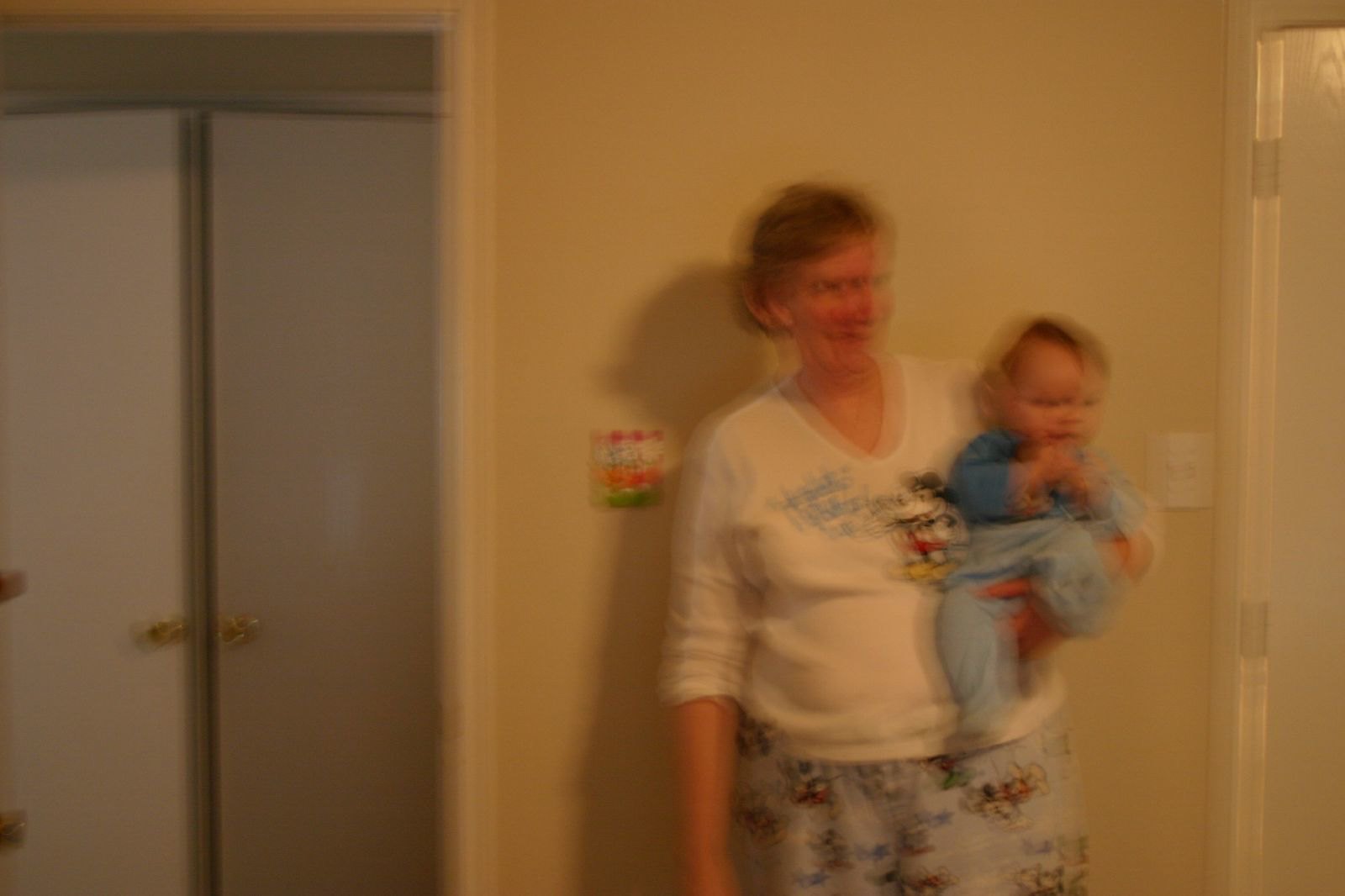In this exceptionally blurred vintage-style photograph, we are presented with a horizontally-oriented image capturing an intimate indoor scene. A woman, leaning against a beige-colored wall, cradles a baby in her arms. Despite the blur, the woman is discernible by her white long-sleeve V-neck shirt, with the sleeves pushed up to her elbows. She faces slightly forward, her gaze directed towards the lower right. The baby's age appears to be around four or five months, adorned in blue bottoms and a dark blue long-sleeve top, with its tiny arms reaching towards its mouth, making it difficult to determine the baby's gender. To the left of the woman are tall, white pantry-like cabinets that stand out starkly against the background. On the right side of the photograph, an open doorway is partially visible, adding depth to the scene. The overall blur creates a double-vision effect, making the detailed features of the subjects nearly indiscernible, contributing to the photo's nostalgic atmosphere.